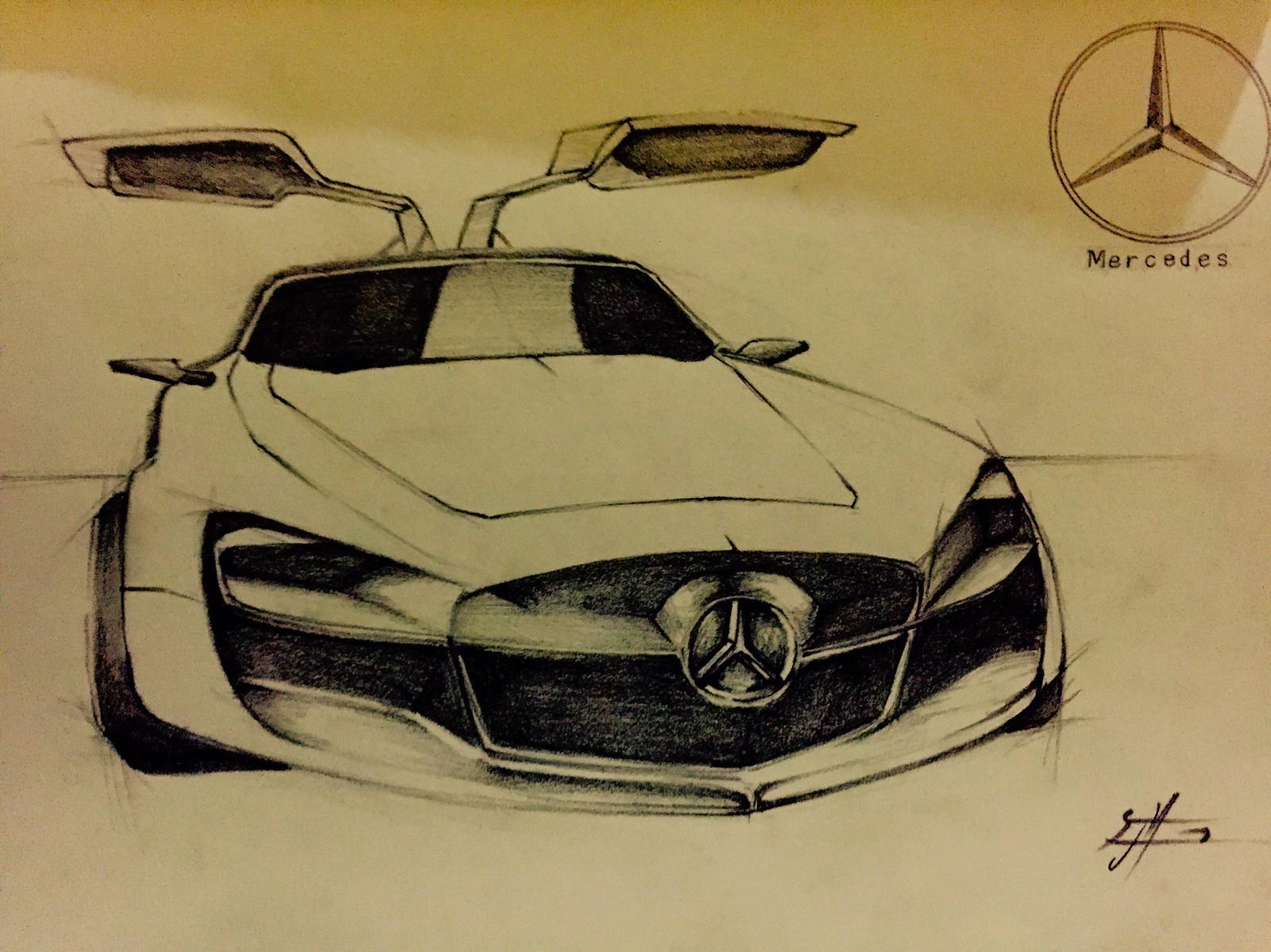This detailed sketch depicts a classic Mercedes car, meticulously drawn on typical computer paper that has yellowed with age, adding a vintage touch. The prominent Mercedes logo adorns the top right corner, complete with the iconic three-pointed star within a circle. The front view of the car dominates the illustration, showcasing the emblematic Mercedes badge on the vehicle's grille. The car's hood is portrayed as distinctly flat, leading up to a windscreen shaded in black with intricate gray highlights to suggest reflective lighting.

A striking feature in this sketch is the car's distinctive gull-wing doors, which open upwards like rabbit ears, adding a dynamic sense of elegance and innovation. Each door includes side mirrors, contributing to the detailed realism of the drawing. At the base of the image, partial views of the car's black tires are visible, grounding the vehicle in its entirety. This detailed artwork captures the essence and luxury of the Mercedes brand through both design and meticulous detail.